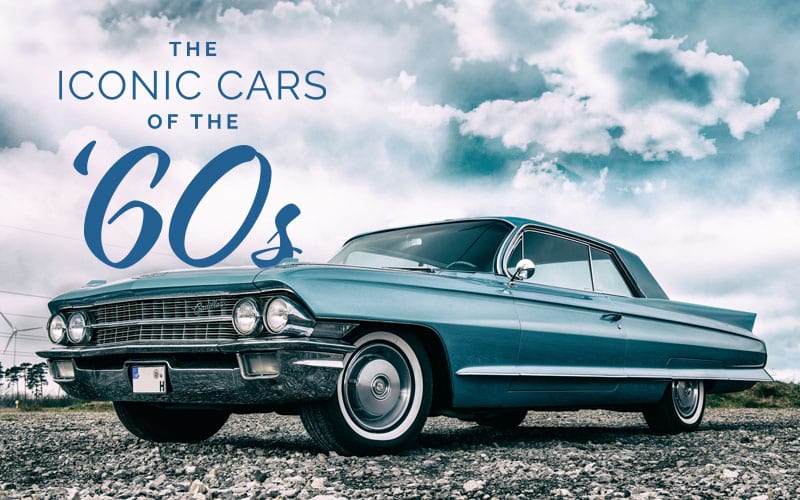This image showcases a teal-colored, sporty car parked at an angle on a gravel surface composed of small black and white stones. The car, representing an iconic model of the 60s, features a single door on the driver's side, visible from the front and side view of the vehicle. Notable details include whitewalled wheels with silver rims, a silver grill, a chrome bumper, and a rear wing. The image is taken from a ground-level angle, which hides the top of the hood. In the upper left corner, "the iconic cars of the 60s" is written in blue text. The background includes white clouds in a teal sky, accompanied by light gray electric lines and windmills.